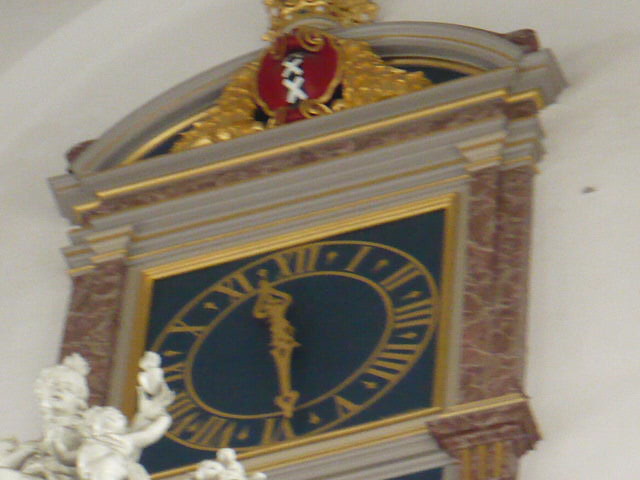This color photograph features an ornate clock affixed to a light gray wall. The clock, appearing to be built into a structure reminiscent of the top of a doorway, showcases a round face encased within a gold frame. This frame is accentuated with two vertical columns, one on each side, which give the clock a grand appearance. The face is decorated with gold Roman numerals and matching gold hands, indicating the time as 11:30.

At the top of the clock, there is a fanciful arch or crescent shape decorated in silver and gold. At the center of this arch, a red circular adornment displays two white "X" markings, one above the other. Additionally, the clock's overall design integrates a combination of gold and marble-like brown textures, enhancing its luxurious aesthetic. The intricate detailing of the frame and embellishments underscores the clock's classical elegance, making it a striking wall-mounted timepiece.